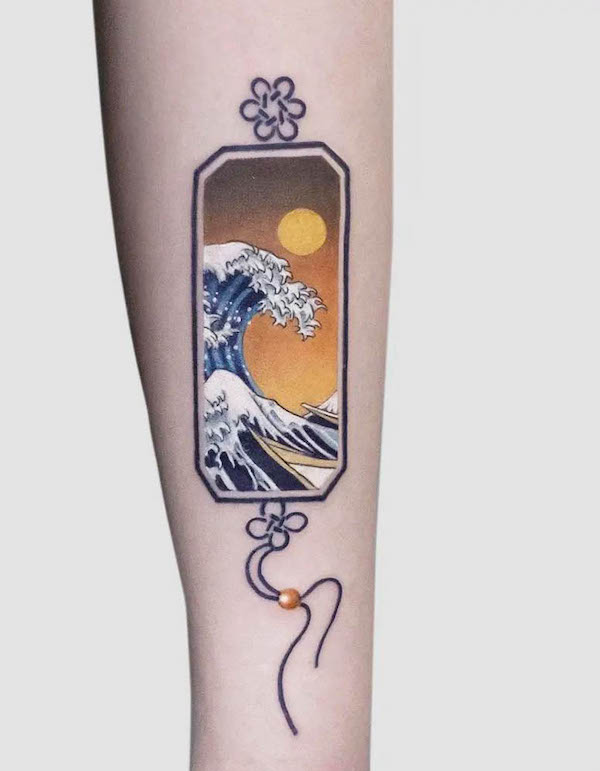The close-up image showcases a detailed tattoo on a person's pale forearm against a white background. The tattoo features an elongated, rectangular design with slightly curved edges, creating an almost octagonal shape. Within this geometric frame, a large, powerful wave is depicted rising from the left side, its crest dark blue with white foamy tips, transitioning to a lighter blue at its base. The backdrop of the wave is a vibrant orange sunset with a glowing yellow sun, casting a warm hue over the scene. At the bottom edges of the wave, the tips of two small boats or canoes are barely visible, adding a sense of scale to the monstrous wave. Above the main wave scene, a black flower is illustrated with intricate detailing, and a similar black flower is positioned below the image, each adorned with wavy strings that extend from their base and converge into a small, brown button-like design, creating a harmonious balance within the overall tattoo.